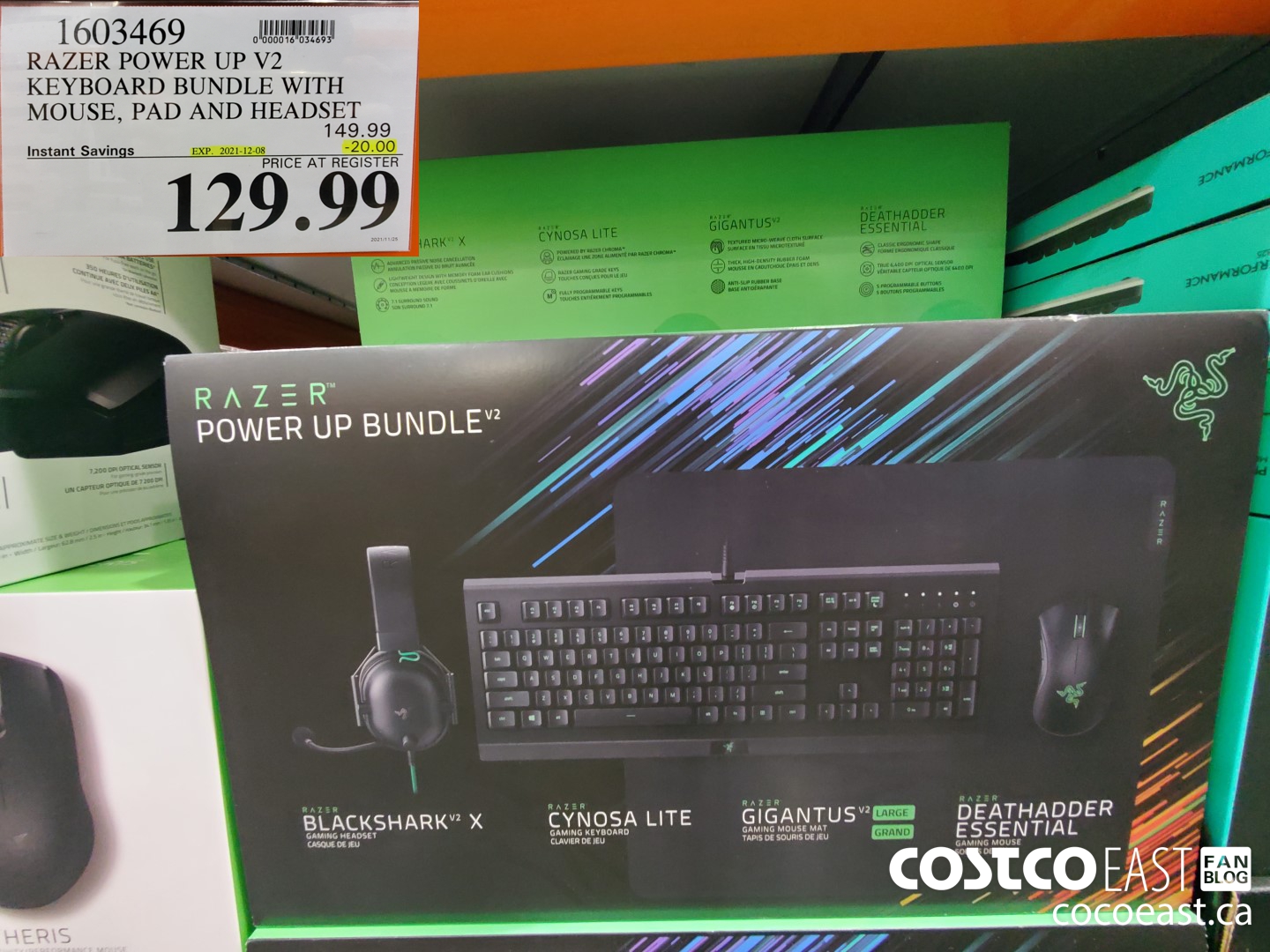The image depicts a retail shelf featuring a prominently displayed Razer Power Up V2 keyboard bundle. The bundle includes a keyboard, Razer BlackShark V2 X headphones, and a mouse, all neatly packaged in a single box. Attached to the box is a price tag that reads "Razer Power Up V2 Keyboard Bundle with Mouse Pad and Headset $149.99," with a highlighted discount of "$20," bringing the total to "$129.99." This special offer is labeled as "instant savings." The tag's barcode number is 1603469.

The boxed bundle is placed on an orange shelf that belongs to a retail store, likely Costco, as indicated by a nearby mention of "Costco East" and a fan blog URL "CostcoEast.ca." Surrounding the Razer bundle, there are other boxes containing laptops and computer mice. The shelf is well-organized, making it easy for customers to identify the product and its discounted price.